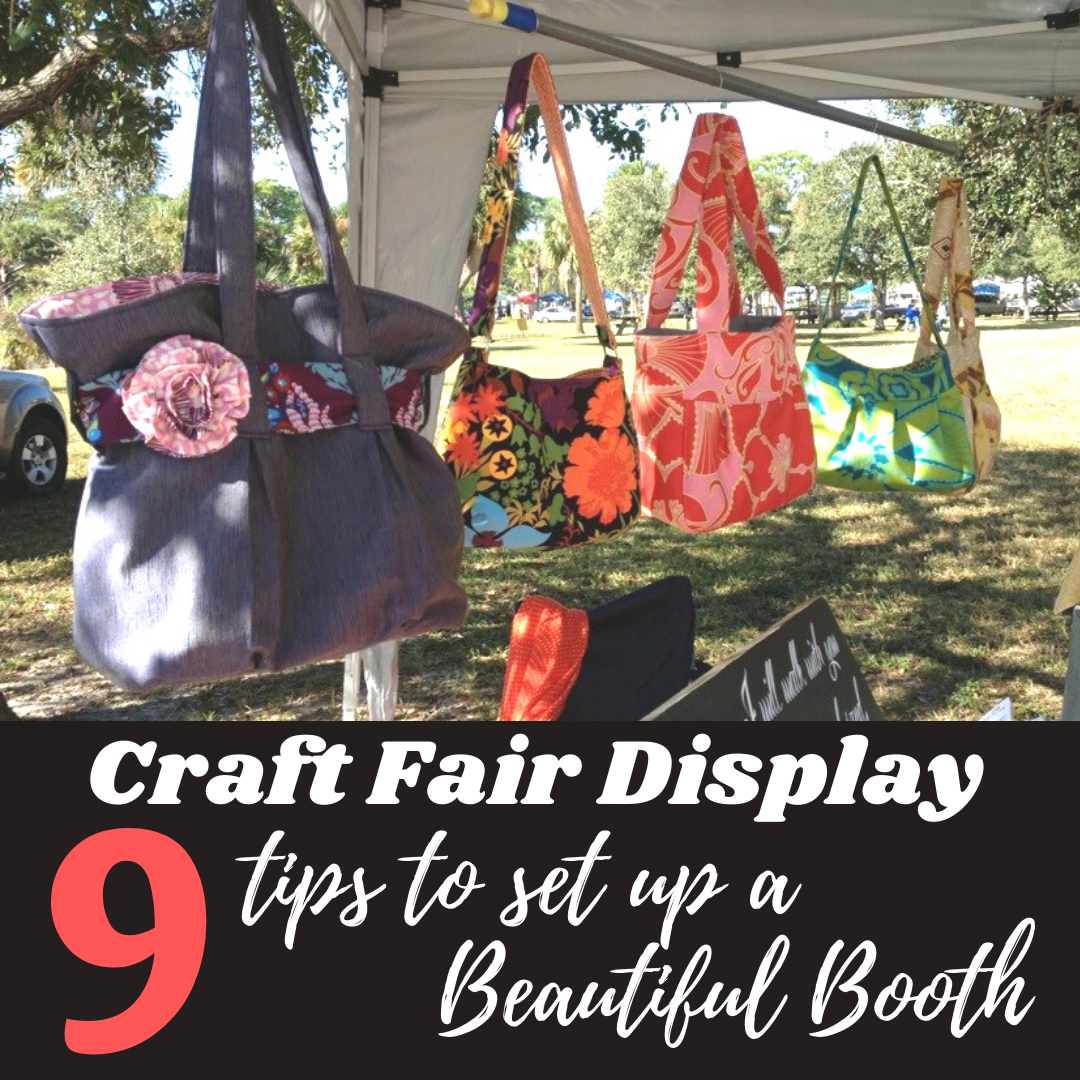The photograph depicts an eye-catching craft fair display set up outdoors under a folding tent with overhead bars. The scene shows a vibrant assortment of handmade handbags suspended from the bars, with an array of colors and patterns. A prominent, black banner with white text at the bottom reads "Craft Fair Display," while additional white cursive text spells out "Tips to Set Up a Beautiful Booth," accompanied by a large red number nine, indicating a listicle or guide.

The handbags are vividly described: the largest is gray accented with pink; another features a floral pattern with striking orange flowers; further along, a bag is adorned in red and pink hues, followed by a green and blue one, and finally, a beige bag with hints of yellow and brown. The bags range from geometric to floral designs, showcasing a wide variety of craftsmanship.

The booth itself is well-integrated into the surrounding environment, with grass underfoot and trees visible in the background, suggesting a park-like setting. Additional elements include a chalkboard and a chair within the tent, and the partial view of a car on the left side. The overall ambiance is bright and sunny, with the booth comfortably shaded, emphasizing the inviting atmosphere of the craft fair.